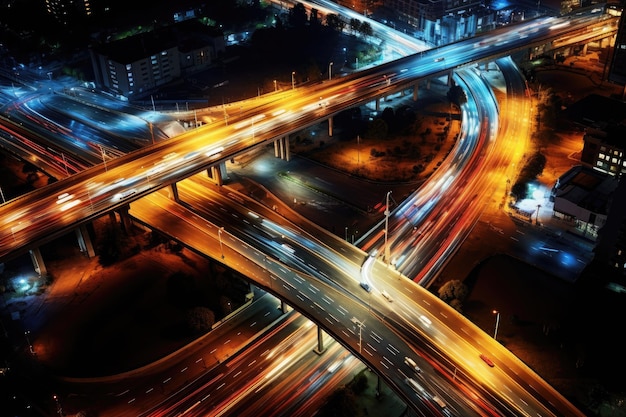This nighttime bird's-eye view captures a complex, multi-tiered highway interchange, reminiscent of what is commonly referred to as Spaghetti Junction. Numerous highways stack above each other, illuminated by streaks of blue and orange lights, giving an impression of motion as the cars speed through the intersection. The top-most highway stretches from the middle left to the upper right corner, while another beneath it runs from the upper middle left towards the bottom right. A third highway starts at the bottom left, ascends towards the right, then curves back to the left, exiting the image in the middle of the top. The surrounding cityscape is dotted with dimly lit streets, scattered buildings, and sparse vegetation, blending into the intricate network of the elevated highways.